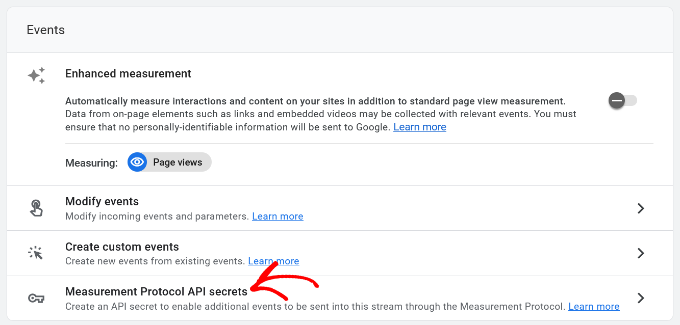In the image, a webpage from a website is displayed, showcasing various categories related to event measurement. At the top, the header reads "Events," under which several options are listed. One notable section features a small sparkly logo on its left side and is labeled "Enhanced Measurement." This section explains that automatically measuring interactions and content on your site, in addition to standard page view measurement, is possible. It mentions that data from on-page elements such as links and embedded videos may also be collected; however, it emphasizes the importance of ensuring that no personally identifiable information is sent to Google. Currently, this function is turned off, allowing a review of user activity on the site.

Below, there is a "Measuring" section listing page views, followed by a dropdown titled "Modify Events." This dropdown, which can be expanded for more details, allows modifications to incoming events and parameters and offers a link to learn more about it. 

Further down, another expandable section titled "Create Custom Events" is visible, providing additional learning resources. 

Lastly, the "Measurement Protocol API Secrets" section, highlighted with a red arrow, instructs users to create an API secret to enable sending additional events to the stream via the measurement protocol, accompanied by a link for further information. 

Overall, the webpage guides users on how to effectively utilize the site’s features to enhance their knowledge and improve the experience for their visitors.